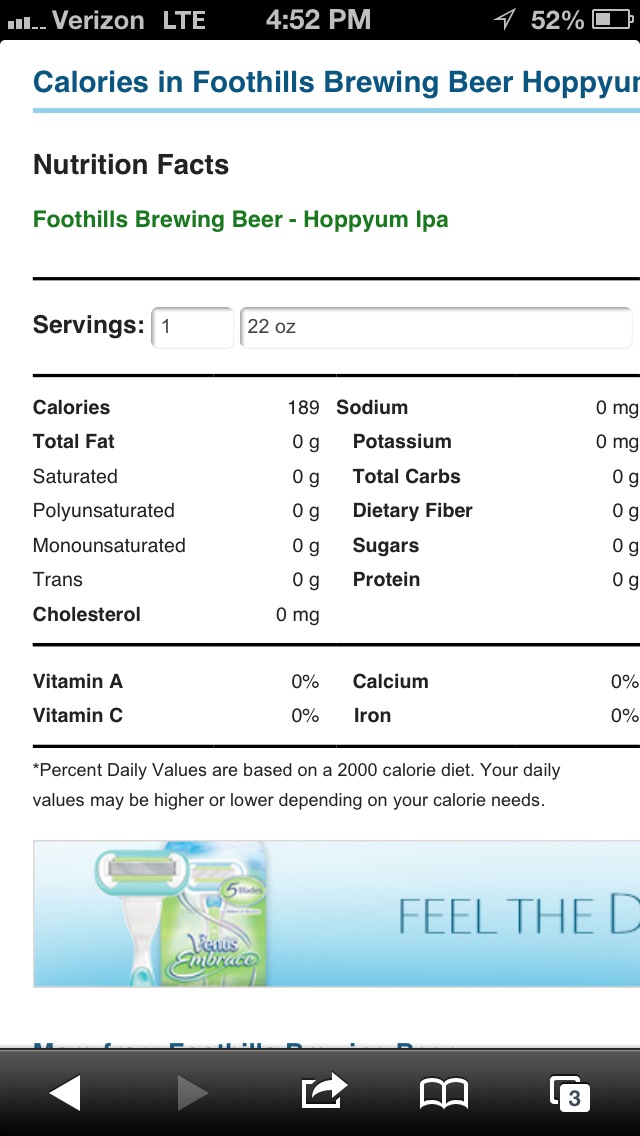The image appears to be a screenshot taken on a Verizon smartphone, as indicated by the black status bar at the top showing "Verizon LTE," the time "4:52 p.m.," and the battery charge at "52%." The following lines provide detailed nutritional information for a product described as "Foothills Brewing Beer - Hoppyum IPA."

An extensive nutrition facts section highlights:

- **Servings**: 1 (22 ounces)
- **Calories**: 189

All the following values are listed as zero:

- Fat (Saturated, Polyunsaturated, Monounsaturated, Trans)
- Cholesterol
- Sodium
- Potassium
- Total Carbohydrates
- Dietary Fiber
- Sugars
- Protein

Further down, the vitamins and minerals, including:

- Vitamin A
- Vitamin C
- Calcium
- Iron

all show values of "0%."

The caption also mentions a standard disclaimer: "*Percent Daily Values are based on a 2,000 calorie diet. Your daily values may be higher or lower depending on your caloric needs.*"

At the bottom of the image, there is a blue rectangle featuring an unclear picture with the text "Feel this" partially visible.